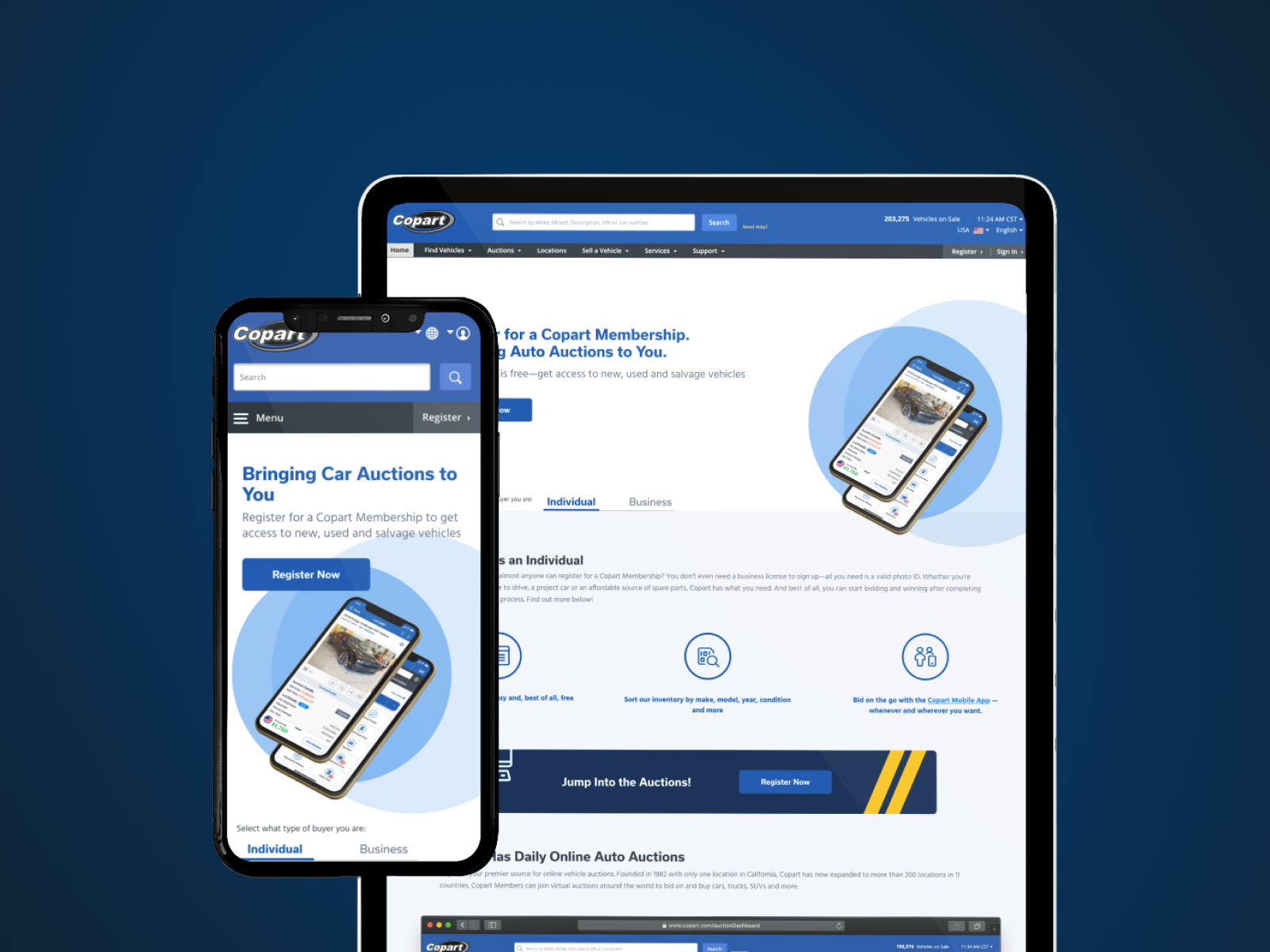The image features a blue background with a prominently displayed smartphone in the foreground. The screen of the smartphone shows the Copart logo, highlighting the brand's identity. At the top, there is a search bar with a magnifying glass icon next to it, indicating the search function.

On the left side of the screen, there is a hamburger menu icon labeled "Menu." Next to the menu, there is a gray square button labeled "Register." Text on the image encourages viewers, stating "I'm bringing car options to you. Register for a Copart membership to get access to new, used, and salvage vehicles. Register now."

Floating above this smartphone is another, smaller smartphone displaying options for selecting the type of buyer, either "Individual" or "Business." There is also a mention of checking the inventory based on make, model, or condition.

A vibrant caption at the bottom advertises the Copart mobile app, which allows users to participate in auto auctions anywhere and anytime. It emphasizes the ease of use with, "Play on the go with the Copart mobile app whenever and wherever you want. Jump into the options. Register now. Daily online auto auctions, merchandise for only vehicle auctions."

Historical context is provided, stating that Copart was founded in 1982 with a single location in California and has since grown to more than 200 locations globally. Members have the opportunity to join virtual auctions worldwide to bid on a variety of vehicles, including Lexus, and more.